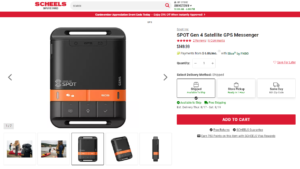The image shows a detailed screenshot from the Scheels website. At the top of the page, there's a red banner with the word "SCHEELS" prominently displayed in bold, all-capital letters. To the right of the banner, there's a search bar accompanied by a red magnifying glass icon. Some text outside the search bar is present but appears extremely blurry and unreadable.

Beneath the red banner, the background transitions to white. In the center-right area of the banner, there's additional white text, but it is also too blurred to decipher. Below this section, the layout includes a central product display with navigation arrows on either side, indicating the option to view multiple images.

The main product showcased towards the left of the screen appears to be a black plastic box. Below this product image, there's an orange banner or line. Additionally, there are four or five smaller images illustrating the product's various uses and positions.

On the right side of the product image, the text reads "Spot Gen3 Safe Flight GPS Messenger," followed by a five-star rating. The price information is present but heavily blurred and not readable. There's also a quantity selector showing "Quantity: 1" with plus and minus buttons for adjustment.

Further down, three distinct rectangles feature graphics with accompanying text beneath them, although the specifics are unclear. Finally, there's a prominent "Add to Cart" button with white text on a red background, signifying the call-to-action for purchasing the product.